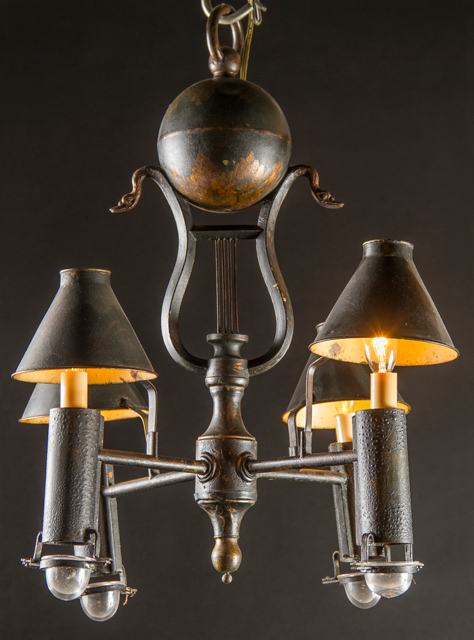This photograph captures an intricate, antique chandelier suspended from a hook against a black background. The fixture begins with a ball ornament at the top, crafted from a blend of copper and dark-colored metal. Beneath the ball, an ornate u-shaped piece adorned with what appear to be small snake heads supports a central fixture. This fixture features four arms extending outwards, each holding a rod-shaped support for candle-like bulbs, which are sheathed in small black, upside-down cone-shaped lampshades. All four bulbs emit a warm yellow glow, enhancing the chandelier's patina brass appearance with shades of copper and dark grey. The base of the chandelier contains a small bulb, completing its elegant, old-world charm.